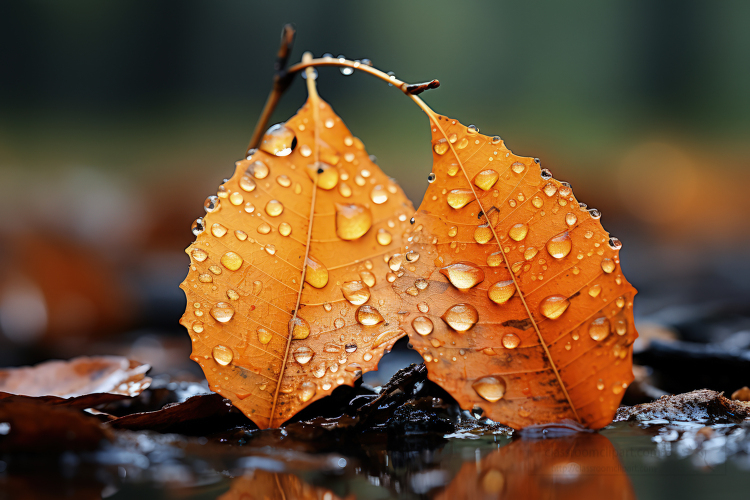This high-resolution outdoor photograph captures an intimate and detailed view of two small autumn leaves connected by a delicate twig. The leaves, which are an orange-yellow with toothed edges, are covered in glistening water droplets from recent rain or morning dew. Their tips touch a small puddle of water below, which reflects the leaves back, enhancing their vibrant color and texture. The background of the image is artistically blurred, composed of soft shades of green and orange, providing a subtle but complementary backdrop. Scattered around the main leaves are additional fallen leaves and natural detritus. The photograph’s exceptional clarity and focus highlight every vein within the leaves, potentially marking it as a professional piece worthy of wildlife photography awards or features in prominent nature magazines.